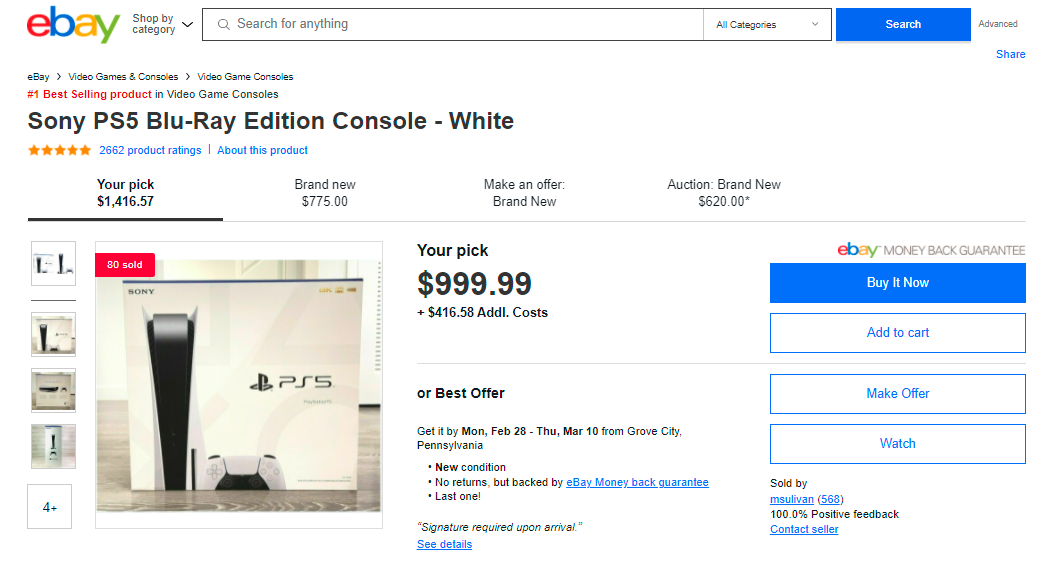Here's a refined and detailed caption for the provided screenshot:

---

The image shows a screenshot from eBay's website. At the top left corner, the distinctive eBay logo is visible with its iconic red, blue, yellow, and green text. Directly below this, the site offers a "Shop by category" option in white text. A search bar follows that allows users to browse "All Categories," with a blue-highlighted search button next to it. To the right of the search bar, the name "Vance" appears in blue text.

The main section of the screenshot focuses on the listing for a video game console. The hierarchy of categories is displayed in black text on a white background: "eBay," "Video Games & Consoles," "Video Game Consoles." A prominent red font announces "Number one best selling product." Below this, in black text, the listing reads "Video Game Consoles," and specifically details "Sony PS5 Blu-ray Edition Console, White." It has an impressive five-star rating from 2,627 reviewers, highlighted in blue.

The listing features several price options in black text: "Your pick" for $1,416.57 (underlined), with different purchasing options outlined in gray underneath. These include brand new for $775, brand new make an offer, brand new auction starting at $620. An image of a PS5 console in its white box with bold black text is prominently displayed. 

In the upper left of the image is a black square with "84 sold" written in white. Another pricing option is available: "Your pick" for $999 plus $416.58 in additional costs or the ability to make an offer. The estimated delivery timeline ranges from Monday, February 20th to Friday, March 10th, shipping from Grove City, Pennsylvania. The call-to-action buttons offer options to 'Buy it now,' 'Add to cart,' 'Make an offer,' or simply 'Watch' the item.

---